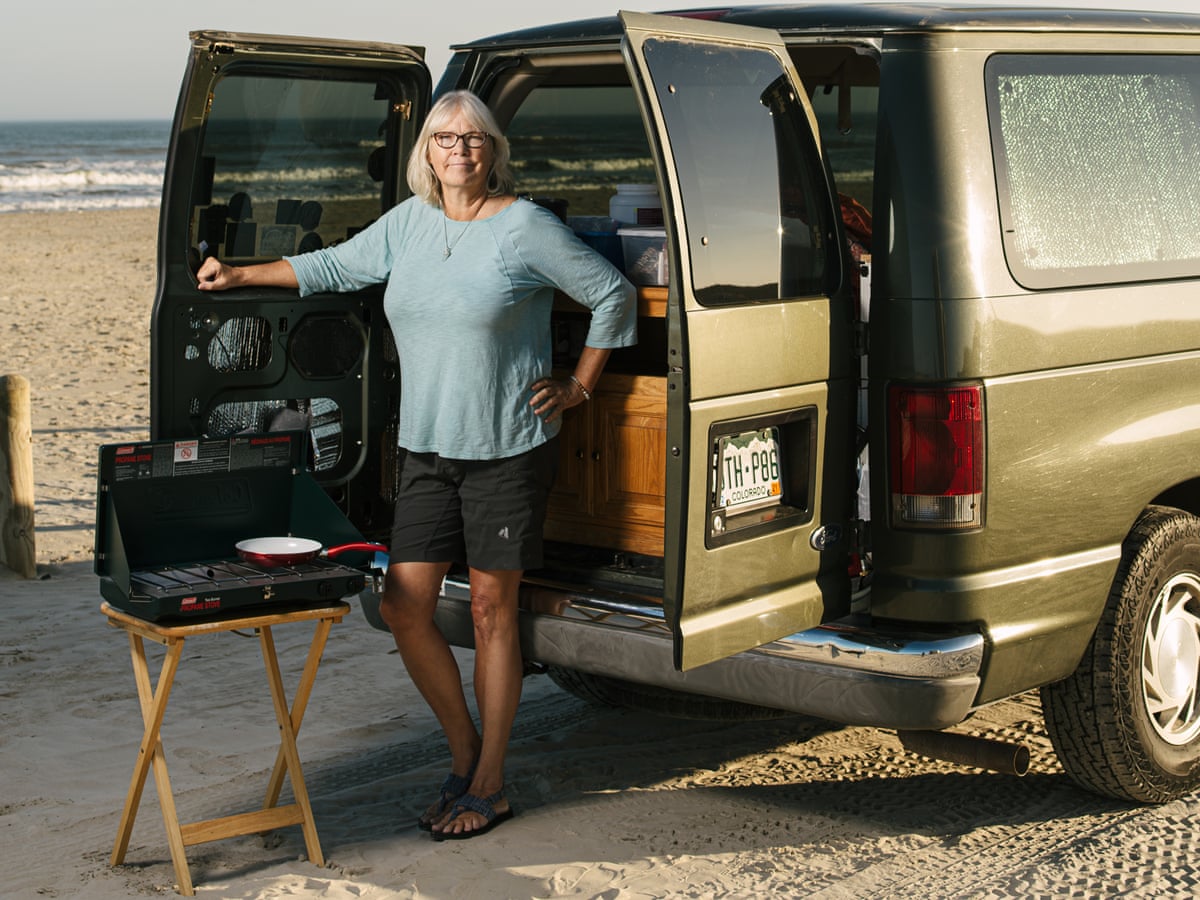The image depicts a middle-aged white woman standing at the back of her metallic gray-brown van, which has a Colorado license plate. She has long white hair, tied in a style that some might describe as a bob with bangs, and she wears glasses. Her attire includes a light blue three-quarter sleeve blouse, black or dark navy blue shorts, and sandals. The van is parked on a sandy beach with the ocean in the background, where gentle waves crest onto the shore.

The van's rear doors are open, revealing what appears to be a makeshift kitchen setup, including cabinets and containers with food. Next to the woman, on the sand, is a small wooden table with a portable two-burner gas stove. On one of the burners sits a bright red and white frying pan. The scene captures a moment of tailgating or camping by the seaside, with the open sky and ocean waves providing a serene backdrop.